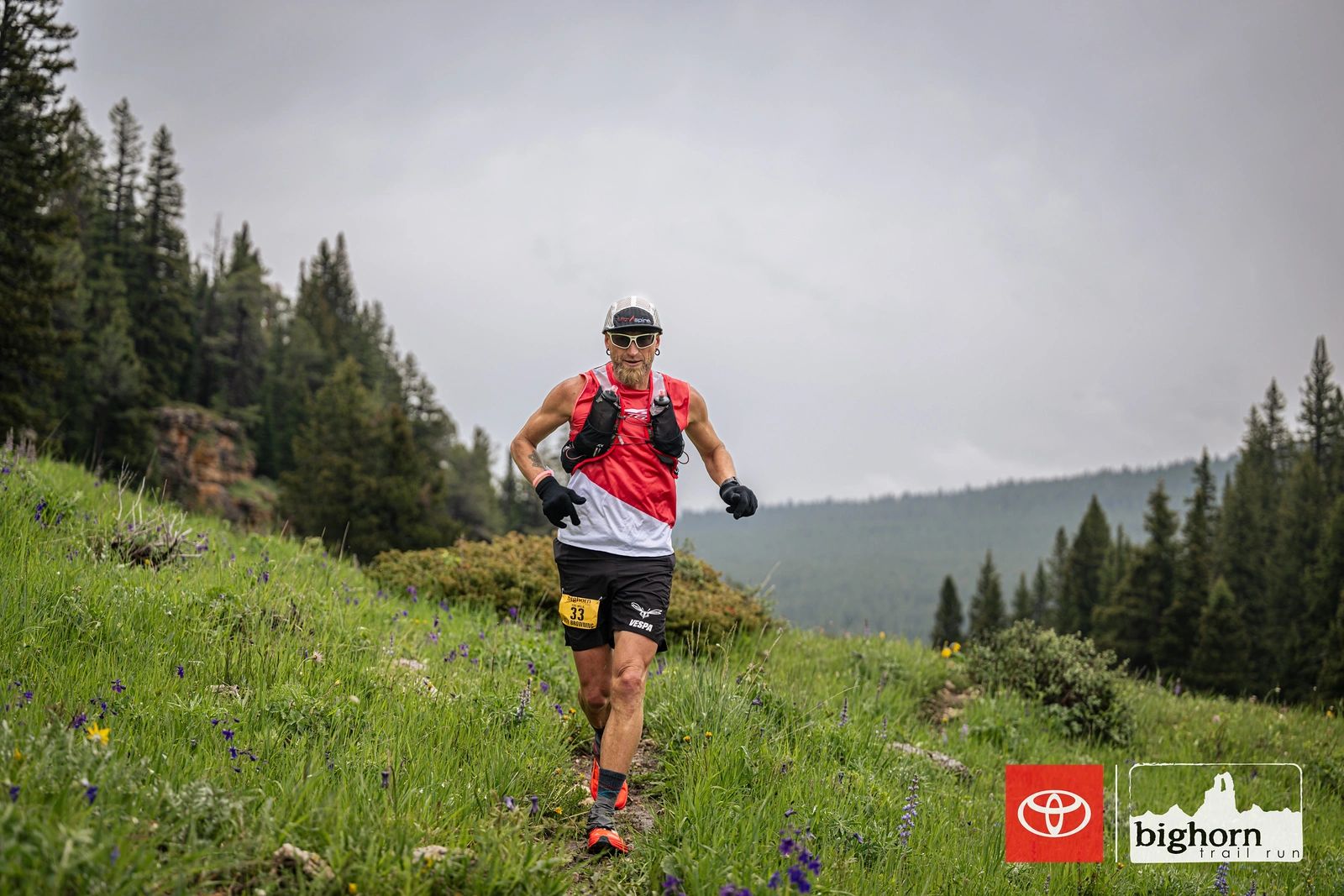A professionally shot, full-color photograph captures a Caucasian male running outdoors on a grassy hillside. The man is wearing black gloves, a white baseball cap worn backwards, silver-framed sunglasses, and hoop earrings. He sports a red and white striped tank top, black running shorts with the number 33 and the word "Vespa" in white, and black and orange running shoes. Additionally, he carries a hydration backpack with a visible tube clipped to his shoulder. The background features a hilly terrain with pine trees in the upper left and right center, a blooming grassy area with flowers, and distant mountains under a gray, clouded sky. The lower right corner of the square image displays the text "Big Horn Troll Run" alongside the red Toyota Motors logo.